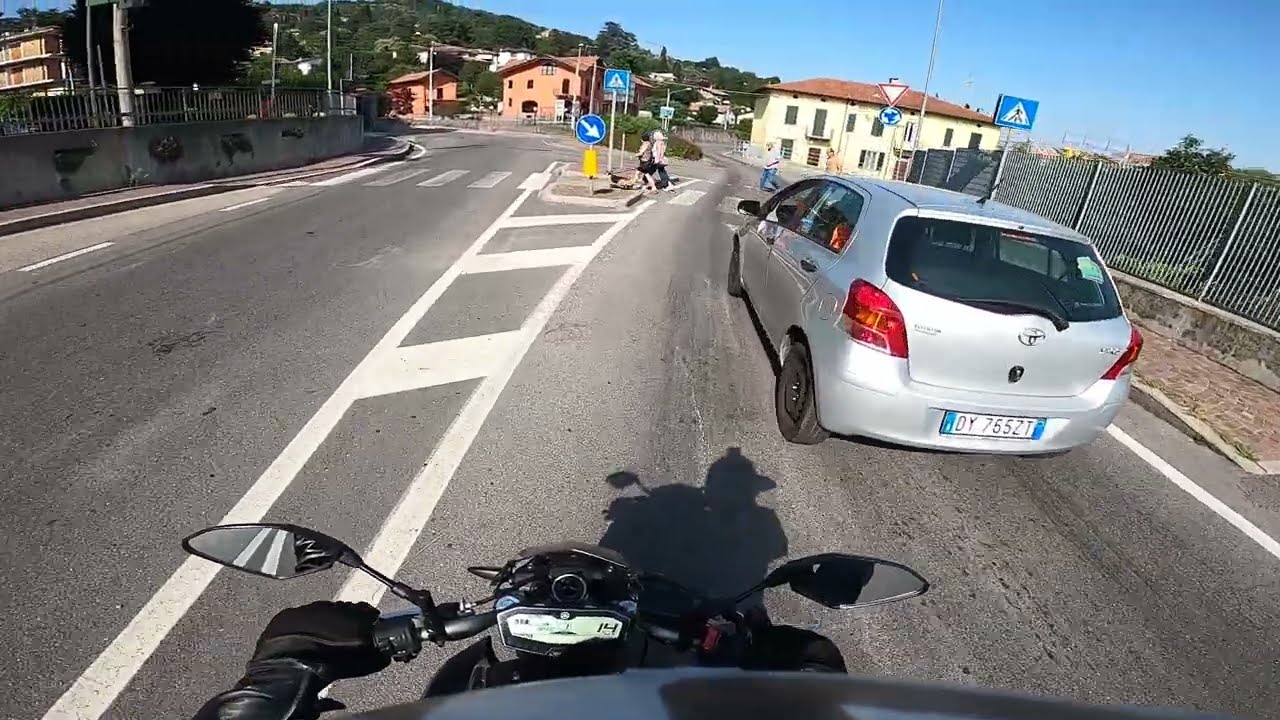In this photo taken from the perspective of someone riding a motorcycle, the observer's point of view showcases the black handlebars and rearview mirrors, with gloved hands gripping the handlebars. The motorcycle is stopped, casting a shadow directly in front. Right ahead is a silver Toyota minivan positioned in the right-hand lane, halted at a crosswalk where four people are crossing. The street has a clear left lane and is marked with white double lines dividing the lanes.

Urban surroundings frame the scene, with buildings in the background—an orange-red structure to the left and a yellow-beige one with a red roof to the right. Further back, the landscape reveals green, tree-covered hills and a clear blue sky above.

On the right side of the image, there's a cobbled brick sidewalk and a blue sign over a fence, along with another blue directional sign at the crosswalk. A two-story yellow building stands nearby. The left side features a concrete sidewalk with a fence on top. Several details like triangular and directional signs add to the urban clutter.